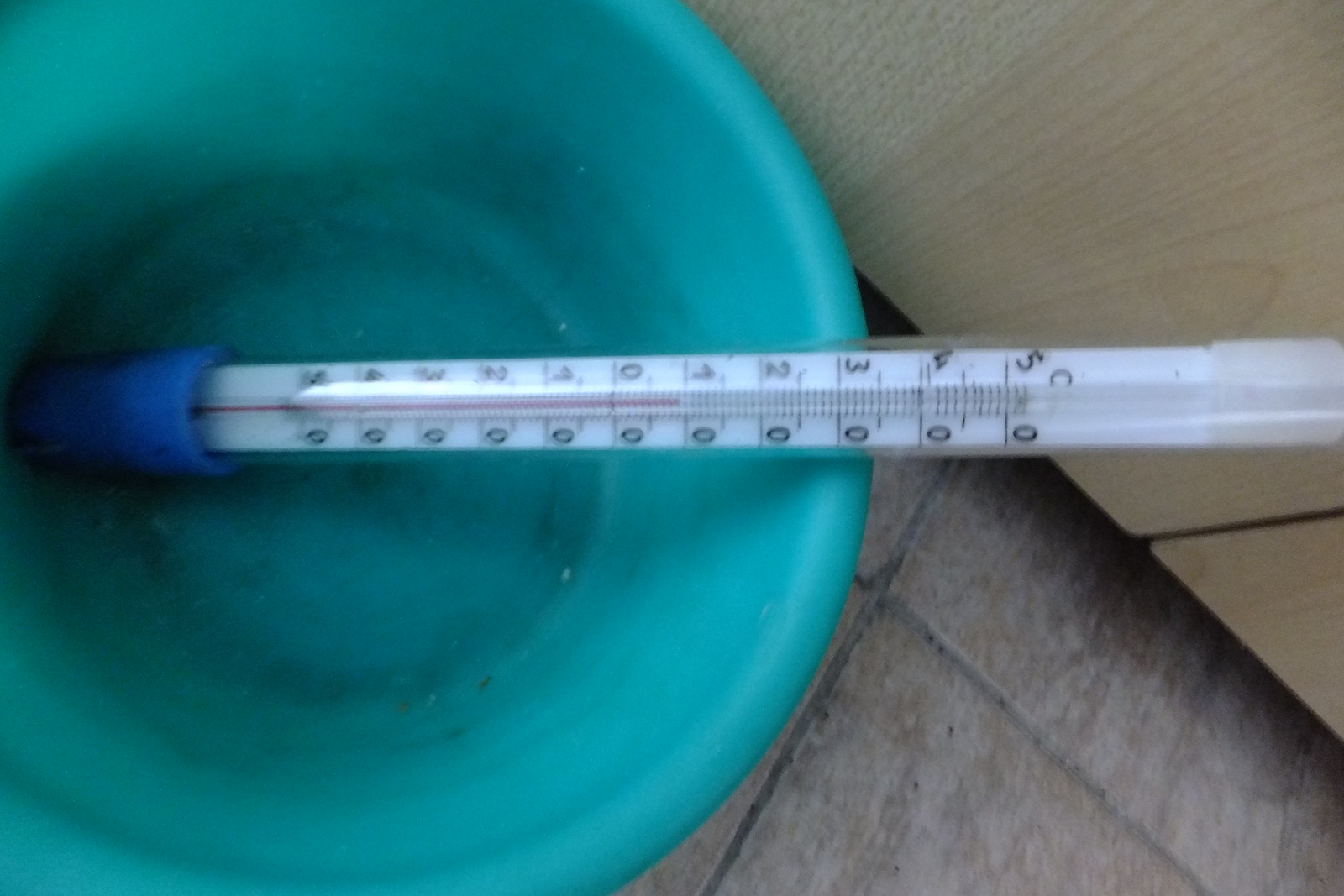This image features a close-up, albeit slightly blurry, photograph of a thermometer. The thermometer is positioned horizontally and spans from left to right within the frame. Notably, it has a distinct blue tip, and its red mercury line rises to just below the one-degree marker on its scale. The scale appears to be marked as 54321012345, suggesting it measures in Celsius. Thus, the thermometer seems to read just under one degree Celsius.

The thermometer is placed inside a blue, plastic-looking bucket, though due to the image's fuzziness, it is difficult to ascertain whether the bucket contains anything. Additionally, the left side of the photo is blurrier than the right, contributing to an overall lack of clarity.

The bucket appears to rest on a floor composed of large square tiles. In the background is a light-colored, beige wooden cabinet, adding context to the scene. The bluish-green, round container holding the thermometer complicates perspective, making the thermometer’s actual size indeterminate. It is challenging to determine the exact nature of what the thermometer is immersed in or its relation to the surroundings based on the information provided.